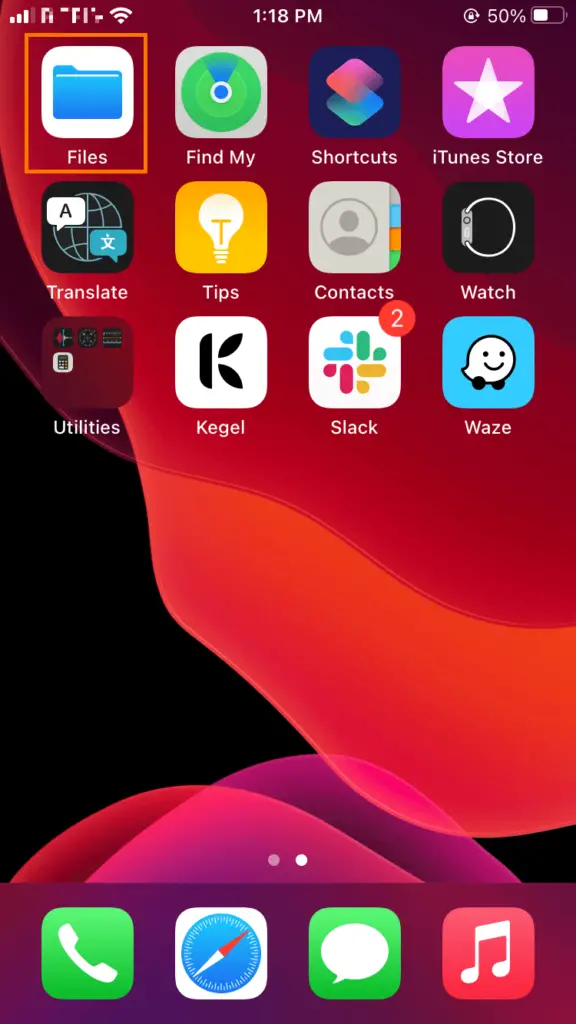Screenshot of a Smartphone's Home Screen: 

The image is a screenshot of a smartphone's home screen, featuring an abstract background with a blend of black, red, and purple hues. At the top of the screen, the status bar displays essential information: from left to right, there is a Wi-Fi icon, signal bars indicating cellular reception, the current time "1:18 p.m.", a battery life percentage showing "50%", and a battery icon.

Below the status bar, three rows of app icons are neatly arranged. The first row includes the following apps:
1. **Files**: Represented by a blue folder icon.
2. **Find My**: Featuring a green circle with a small location icon inside.
3. **Shortcuts**: Symbolized by two overlapping squares.
4. **iTunes Store**: Identified by a pink star on a white background.

The second row consists of:
1. **Translate**: An app icon with a globe and an "A" alongside a Chinese character.
2. **Tips**: Displaying a light bulb with a "T" inside it.
3. **Contacts**: Featuring the standard contacts silhouette icon.
4. **Watch**: Depicted by a simplified drawing of a wristwatch.

The third row contains:
1. **Utilities**: A folder icon that includes four smaller app icons inside.
2. **Kegel**: Identified by a simple “K”.
3. **Slack**: An app with multi-colored hashtag-like icon.
4. **Waze**: Featuring a blue smiley face icon.

This organized arrangement of apps ensures easy access to frequently used functions and services on the smartphone.